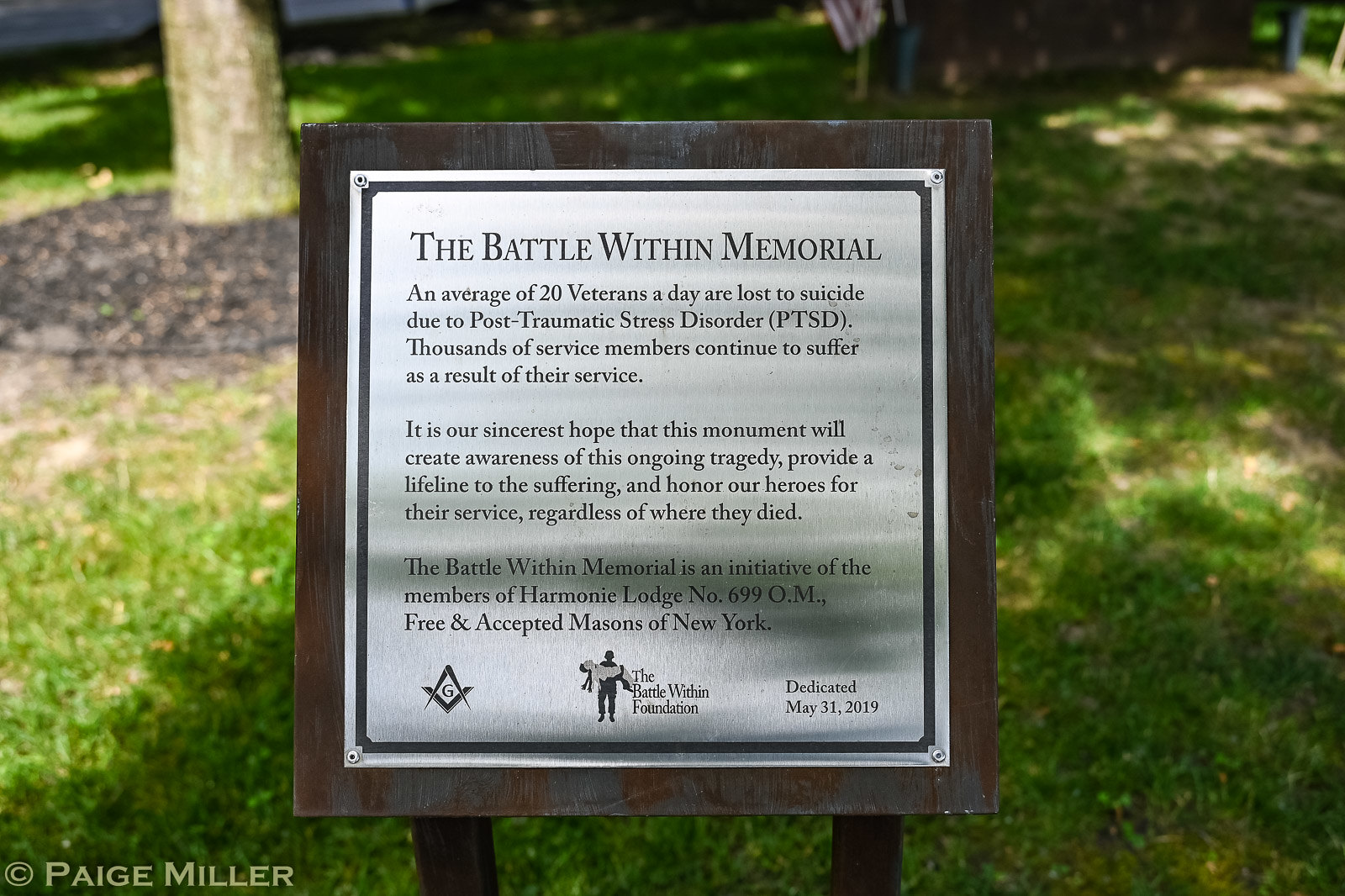This image depicts a rust-colored sign with a silver metal plaque framed in brown, located in a park in New York. The plaque, bolted to the frame, has a black border and features black text on a white background. The top of the plaque reads in capital letters: "THE BATTLE WITHIN MEMORIAL." Below this title, the text details that an average of 20 veterans a day are lost to suicide due to Post-Traumatic Stress Disorder (PTSD), and thousands of service members continue to suffer as a result of their service. The plaque expresses the hope that the memorial will raise awareness about this ongoing tragedy, provide a lifeline to those suffering, and honor the heroes for their service regardless of where they died. 

Additionally, the plaque notes that "The Battle Within Memorial" is an initiative by the members of Harmony Lodge No. 699-OM Free and Accepted Masons of New York. At the bottom of the plaque, there's an illustration of a person holding another person in their arms, associated with "The Battle Within Foundation." The inscription also includes the dedication date: May 31, 2019. The background of the image features neatly landscaped green grass and trees.